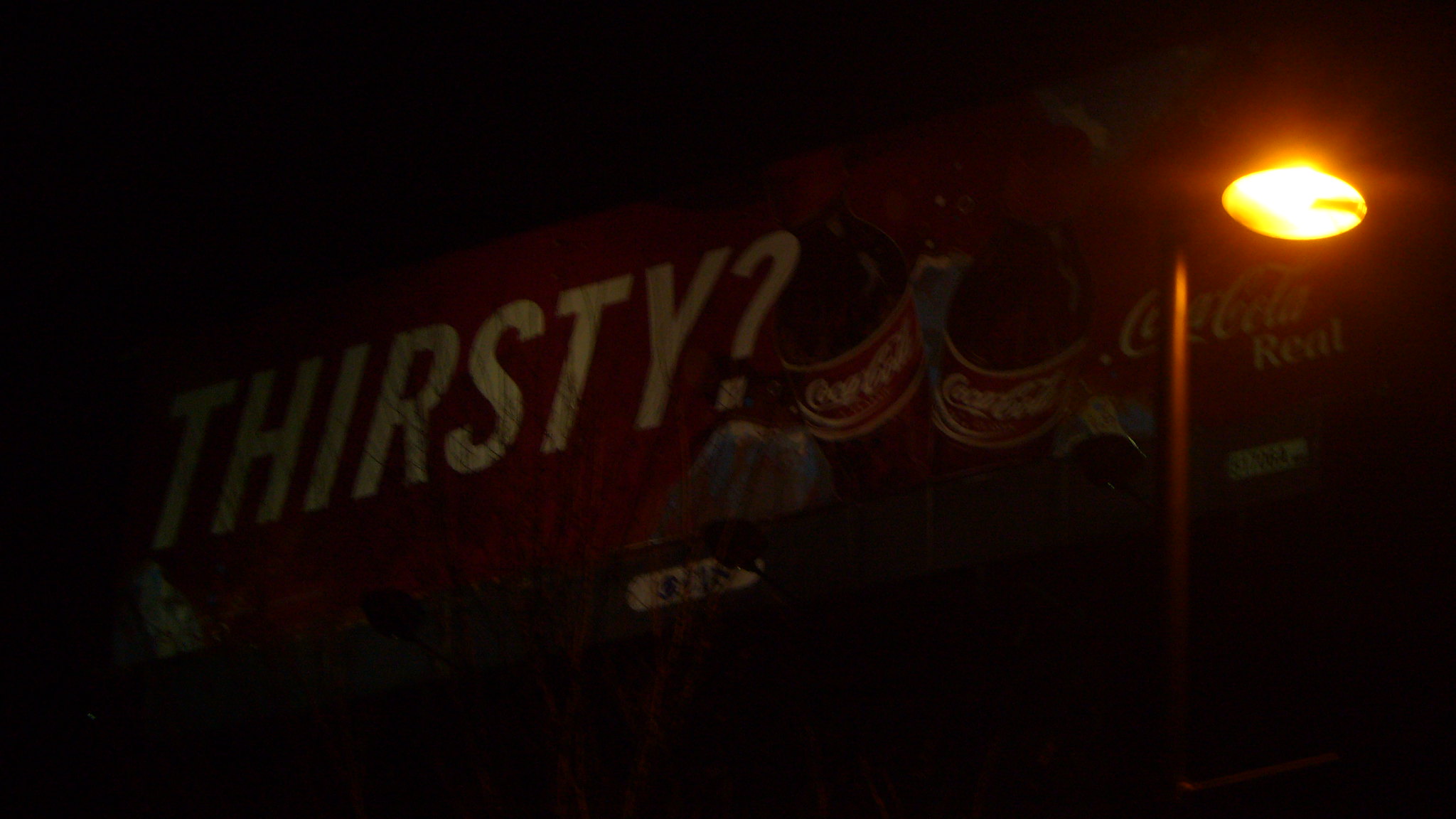This nighttime photograph captures a dimly lit scene dominated by a Coca-Cola billboard. The image quality is not high, contributing to the overall dark and somewhat blurry ambiance. An illuminated streetlamp to the right emits a yellow glow, partially revealing the billboard. The billboard's main feature is the large white text "THIRSTY?" set against a red background. Below the text, there are two vertical Coca-Cola bottles, each adorned with the iconic red label and white cursive branding. A smaller version of the Coca-Cola logo appears on the far right of the billboard, accompanied by the word "REAL" beneath it. The streetlight’s light provides just enough illumination to make out these details, while the rest of the surroundings remain obscured by darkness.